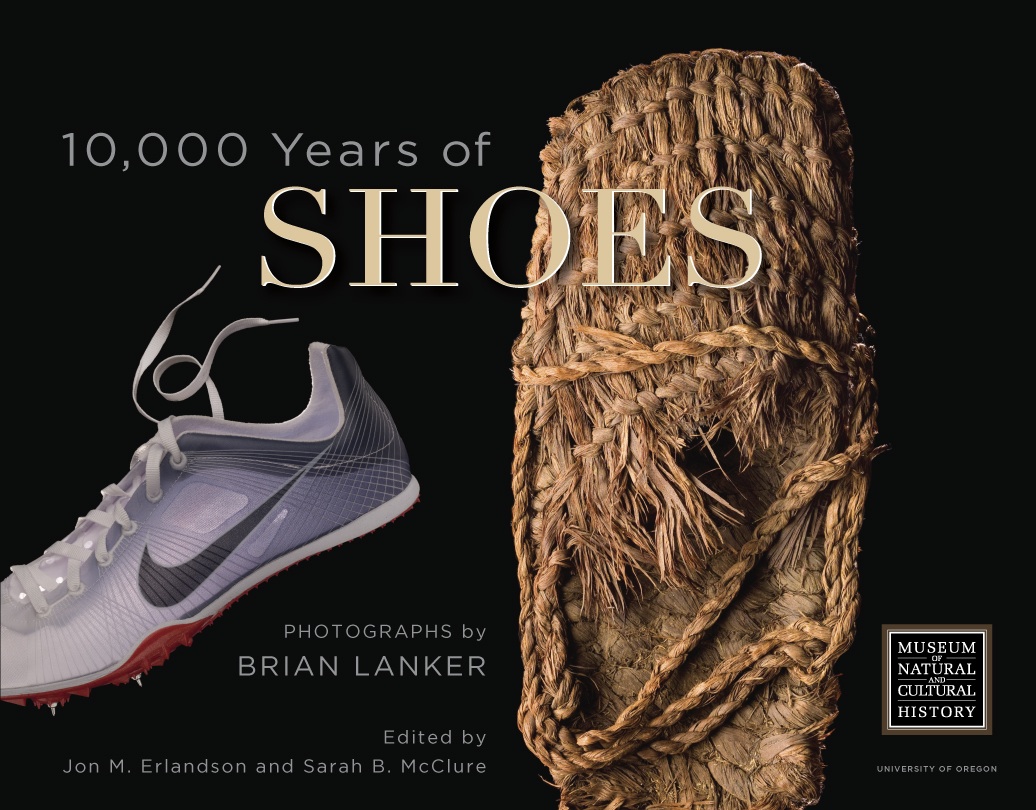The image features a black background with the title "10,000 Years of Shoes" prominently displayed at the top in large white text. Below this title, there is text indicating "Photographs by Brian Lanker" and at the bottom, another text line states "Edited by John M. Erlinson and Sarah B. McClure." 

On the left side of the image, a modern Nike tennis shoe, primarily white with a gray swoosh on the side, is depicted. The shoe appears to float diagonally from the bottom left corner, with its white laces extended upward. The shoe may have spikes on the bottom. 

Contrastingly, on the right side of the image is a primitive, homemade footwear item that resembles a snowshoe, seemingly constructed from dry grass and rope. This historical shoe is a woven design, using thin brown ropes and appears to be a slip-on style.

The image appears to be an advertisement or promotional piece, likely for an exhibition or publication by the Museum of Natural and Cultural History at the University of Oregon.